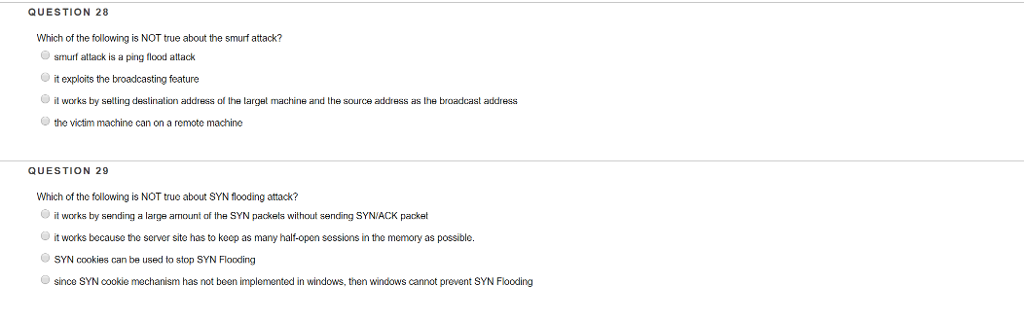The image features a predominantly white screen displaying multiple-choice questions centered around cybersecurity attacks. At the very top, there is a faint black line extending horizontally from left to right. Below this line, the text "Question 28" is displayed in a large, bold font. 

Following Question 28, there's a smaller-font query: "Which of the following is not true about the Smurf attack?" Below this query, there are four grey, large, round bullet points presenting the options:

1. Smurf attack is a ping flood attack.
2. It exploits the broadcasting feature.
3. It works by setting the destination address as the address of the target machine and the source address as the broadcast address.
4. The victim machine can be on a remote machine.

Underneath these options, a faint grey line runs horizontally across the screen, followed by a space, and then another identical faint grey line. Beneath the second line, "Question 29" is displayed in a large, bold font.

The text for question 29 reads: "Which of the following is not true about the SYN flooding attack?" Again, there are four grey, large, round bullet points listing the options:

1. It works by sending a large number of SYN packets without sending SYN/ACK packets.
2. It works because the server side has to keep as many half-open sessions in memory as possible.
3. SYN cookies can be used to stop SYN flooding.
4. Since SYN cookie mechanisms have not been implemented in Windows, Windows cannot prevent SYN flooding.

The clear, structured format along with the consistent use of visual elements like lines and spacing, aid in reading comprehension and visual clarity.